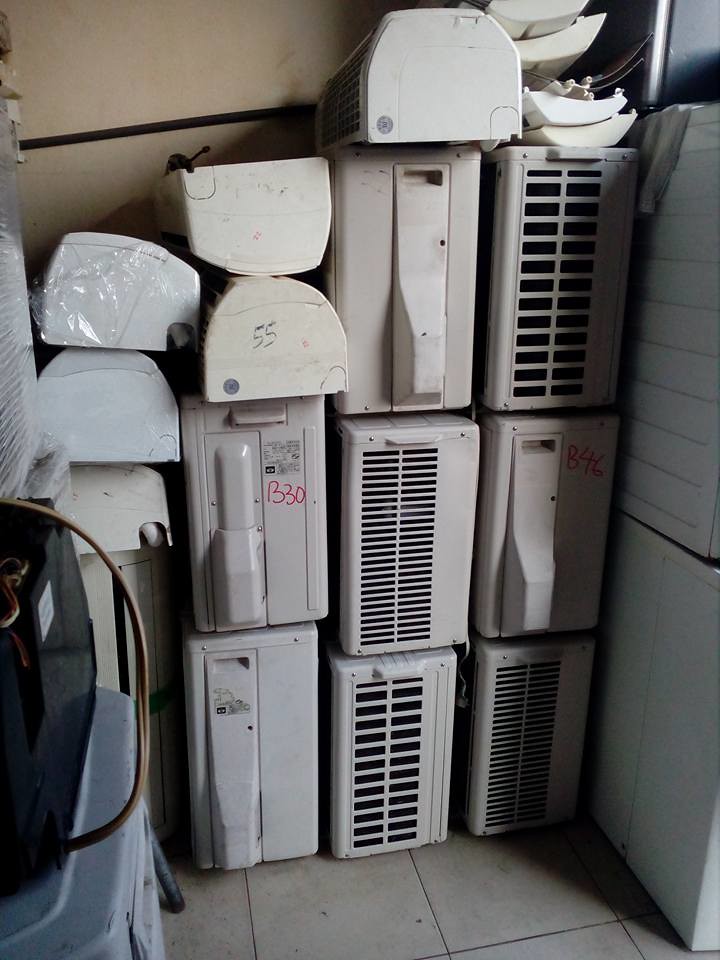The image is a detailed, color photograph capturing various gray, hard-plastic and possibly metal case-like objects, which are meticulously stacked in the corner of a room. The majority of the image is dominated by these rectangular containers, which feature ventilation slits on their sides, suggestive of some electronic equipment, potentially space heaters or other appliances. They are organized into three primary stacks: the left stack is two units high, while the middle and right stacks are three units high each. Some of the containers are marked with numbers and letters in red and black marker, such as "B30" and "55." The cases are stacked on a beige tile floor with dark grout lines, adding texture to the setting. The wall behind is painted beige, contributing to the room's somewhat dingy atmosphere. Additionally, a sliver of another indistinguishable stack is visible to the left, appearing alongside a light blue or gray metal bin with an attached device and cord. On top of the rightmost stack, there are also four lids neatly piled. The photograph is thoughtfully framed in a portrait orientation, capturing the stark and orderly arrangement of these enigmatic items against their muted background.